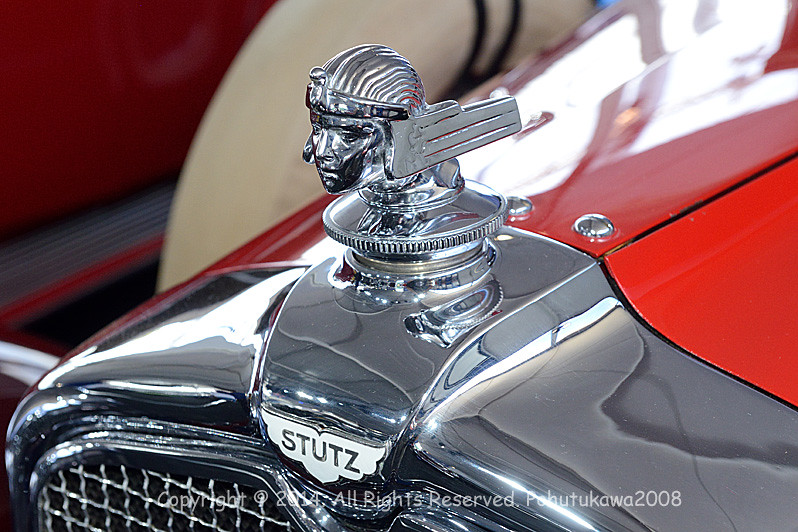This photograph features the hood of a vintage red car with a silver, exceptionally shiny fender. Centered on the hood is an emblem depicting a man's face adorned with a headband, long hair, and other indistinguishable objects. The front fender displays the word 'Stitz' on a white background that contrasts with the silver fender. Additional details include a prominent grill and various knobs and screws protruding from the front, along with marks indicating a trademark or copyright dated 2014, associated with Pabu Tukawa from 2008.